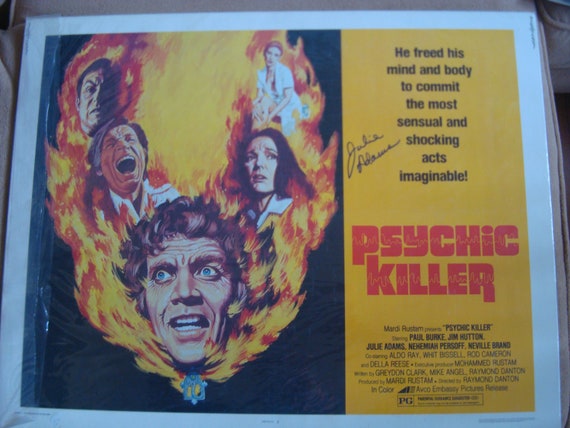This movie poster features a striking visual composition. On the left side, five individuals—three men and two women—are depicted with expressions of shock and fear as they appear to be engulfed by encroaching flames. Their wide eyes and open mouths heighten the sense of terror. On the right side, the poster prominently displays the title "PSYCHIC KILLER" in bold, red capitalized sans serif font. Above the title, a tagline reads in black text: "He tried...". The overall design and fiery elements evoke a sense of suspense and horror, perfectly encapsulating the movie's chilling theme.